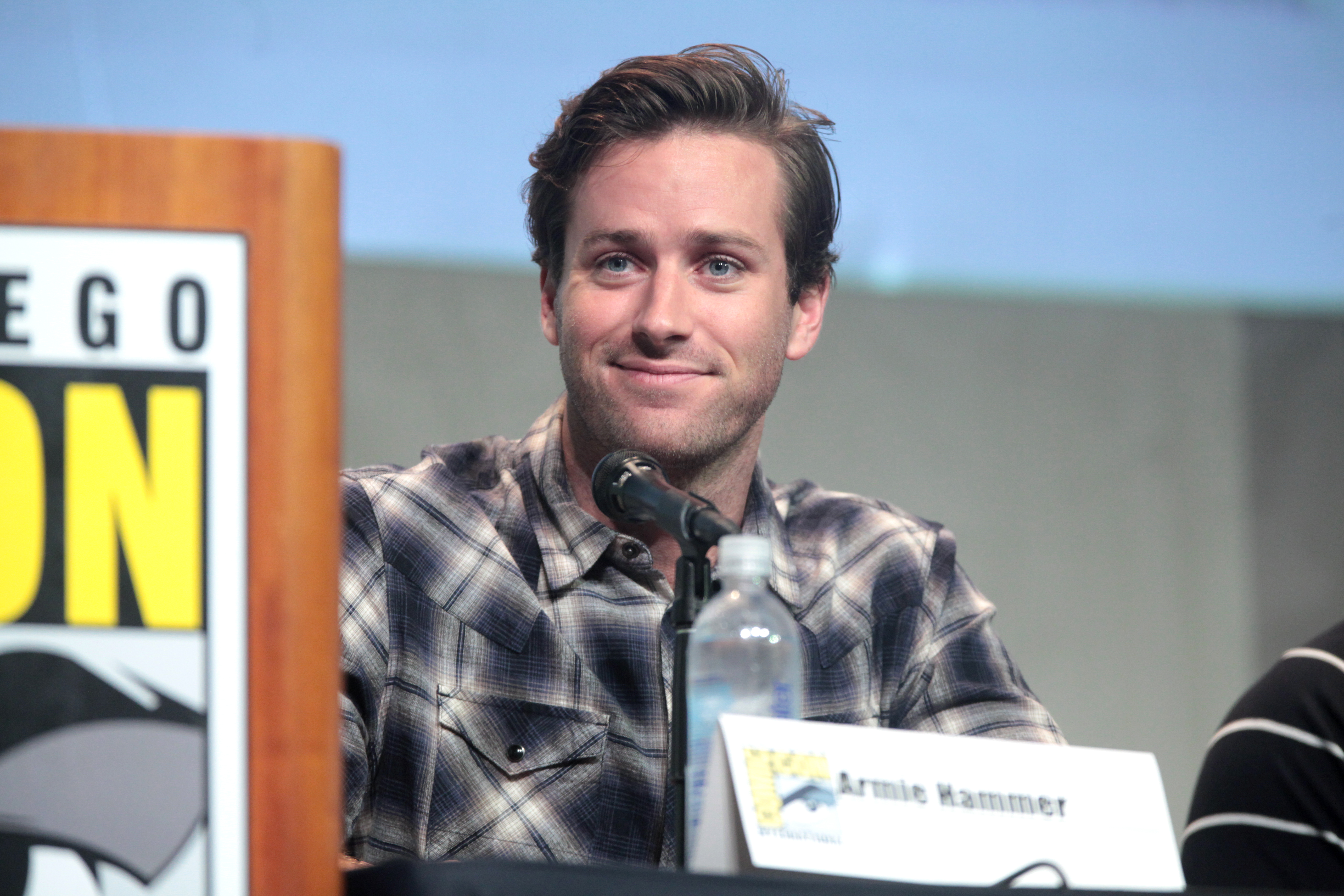This detailed image captures Armie Hammer at what appears to be San Diego Comic Con, sitting behind a table equipped with a microphone and a bottle of water. In front of him, there's a nameplate with his name in white with black letters, alongside a colorful sign featuring black, yellow, and blue details. Armie Hammer, a young white male, has neatly parted dark brown hair, piercing blue eyes, and a thin layer of facial hair. He is clad in a black, grey, and white plaid button-down shirt that exudes a lumberjack vibe. He sports a slight smirk as he looks to the side, possibly engaging with someone nearby. To his right, the corner of a wooden podium is partially visible, and the photo's background transitions from grey to light blue near his head. The scene gives off the distinct atmosphere of a convention, further suggested by another individual seated to Armie's right, identifiable only by their black and white striped sweater.